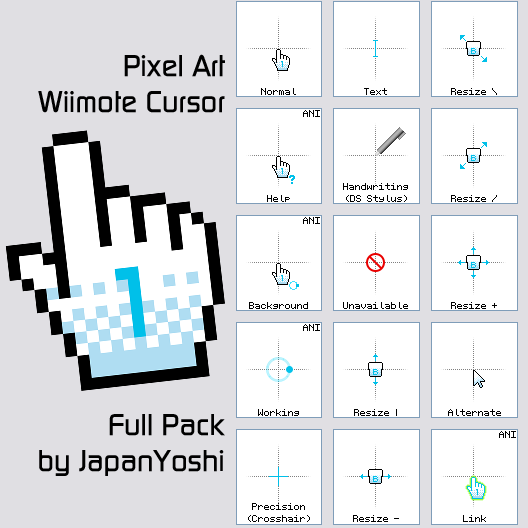The image showcases a preview of a pixel art Wiimote cursor pack titled "Pixel Art Wiimote Cursor," prominently featured is a large pixelated hand, resembling a white glove with a blue number one on the index finger, positioned on the left side along with the text "Full Pack by Japan Yoshi." The background is gray, and on the right half of the picture, there are fifteen smaller white squares, each displaying a different cursor design, complete with labels. These include various functions like Normal, Text, Resize (with blue arrows for different directions), Help (depicted by a hand with a question mark), Handwriting (shown as a DS stylus), Background, Unavailable (displayed as a red stop sign), Working (a blue circle), Alternate (the standard mouse cursor), Precision (a crosshair), and Link (a green hand). This collection seems to be an assortment of customizable cursor options for the Wiimote control, each meticulously crafted in pixel art style.